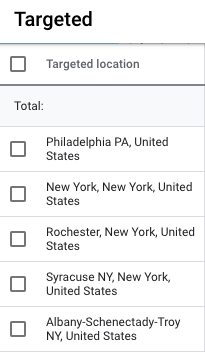The image showcases a user interface screen with a white background, displaying multiple checkboxes accompanied by location labels. At the very top, there is a checkbox labeled "Targeted Location" that is currently unchecked, enclosed between two thin gray lines.

Beneath this, a light gray box with the word "Total" in bold black text is prominently displayed. Below the "Total" box, there are five distinct checkboxes, each paired with a respective location. All checkboxes are in a blank (unchecked) state. The listed locations from top to bottom are:

1. Philadelphia, PA, United States
2. New York, New York, United States
3. Rochester, New York, United States
4. Syracuse, New York, United States
5. Albany, Schenectady, Troy, New York, United States

Each location is meant to represent a selectable option for targeting purposes, but none have been selected as of yet.